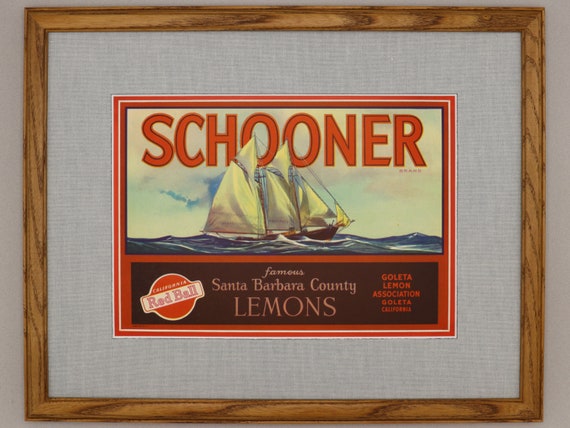This image showcases a dark wooden picture frame, possibly made from pine or fir, featuring a vintage-style advertisement. The frame is bordered by a gray insert that highlights the central illustration of an old wooden schooner with a prominent white sail navigating blue ocean waves. Above the ship in red text is the word "Schooner." The sky in the background is a vivid blue filled with clouds. Below the illustration, there's a detailed label that reads "Santa Barbara County Lemons" with additional text, "Goleta Lemon Association" on a red ball emblem, all within a red border. The label gives the impression of an old product advertisement, specifically for lemons from Santa Barbara, California.